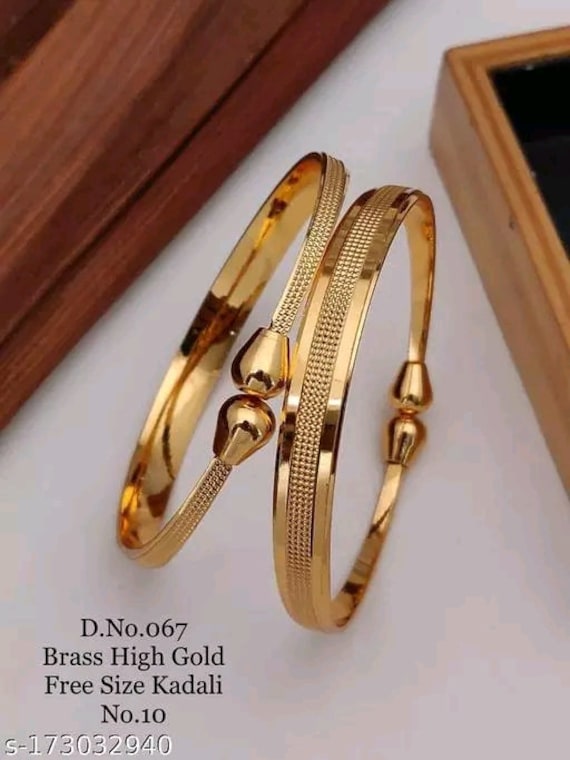This image depicts an advertisement for two intricately designed gold bracelets or earrings made from brass high gold. These jewelry pieces, labeled with the product code "D-NO-067" and described as "free size Kadali number 10," are positioned at the center on a white table, their textured bands showcasing a rougher texture that adds to their aesthetic value. The items are standing upright, seemingly unsupported, creating an elegant visual effect with their reflection visible on the table surface. In the upper left-hand corner, there is a darker wooden trim piece that extends diagonally, while on the right side, there is a wooden frame or container with a black interior, likely used for displaying these jewelry pieces. The bottom left corner contains further product information in black text: "D-NO-067, brass high gold, free size, Kadali number 10, S-173032940." The detailed engravings and unique design elements highlight their sophisticated craftsmanship, making these pieces stand out in the display.